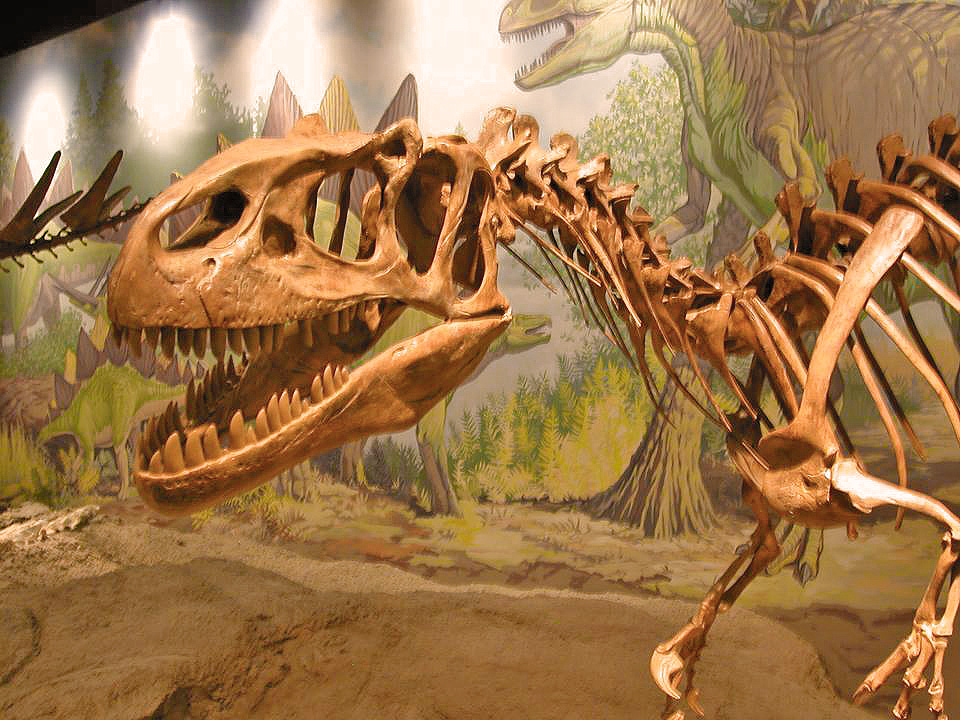The photograph captures an up-close view of a partially assembled dinosaur skeleton, predominantly featuring the skull, neck, and shoulder region, which suggests it might be a Tyrannosaurus rex based on its small arms and predatory features. The fossilized bones are a light tan color, giving a sense of age and preserved history. The dinosaur's mouth is open, displaying an impressive array of fossilized teeth. The backdrop provides additional context, showcasing a hand-drawn or illustrated scene of a prehistoric landscape. This background features a dramatic encounter with a living T. rex, its mouth agape and seemingly in pursuit of a Stegosaurus, whose distinctive spiked tail is partially visible to the left. The illustration behind the fossil includes muted tones of browns, tans, and greens, with hints of black in the upper left, and large trees providing a natural setting. The skeleton appears to be standing on a rocky display, blending into the museum's diorama that integrates both the reconstructed fossils and the vibrant depiction of the ancient environment. This scene vividly brings to life the world in which these magnificent creatures once roamed.